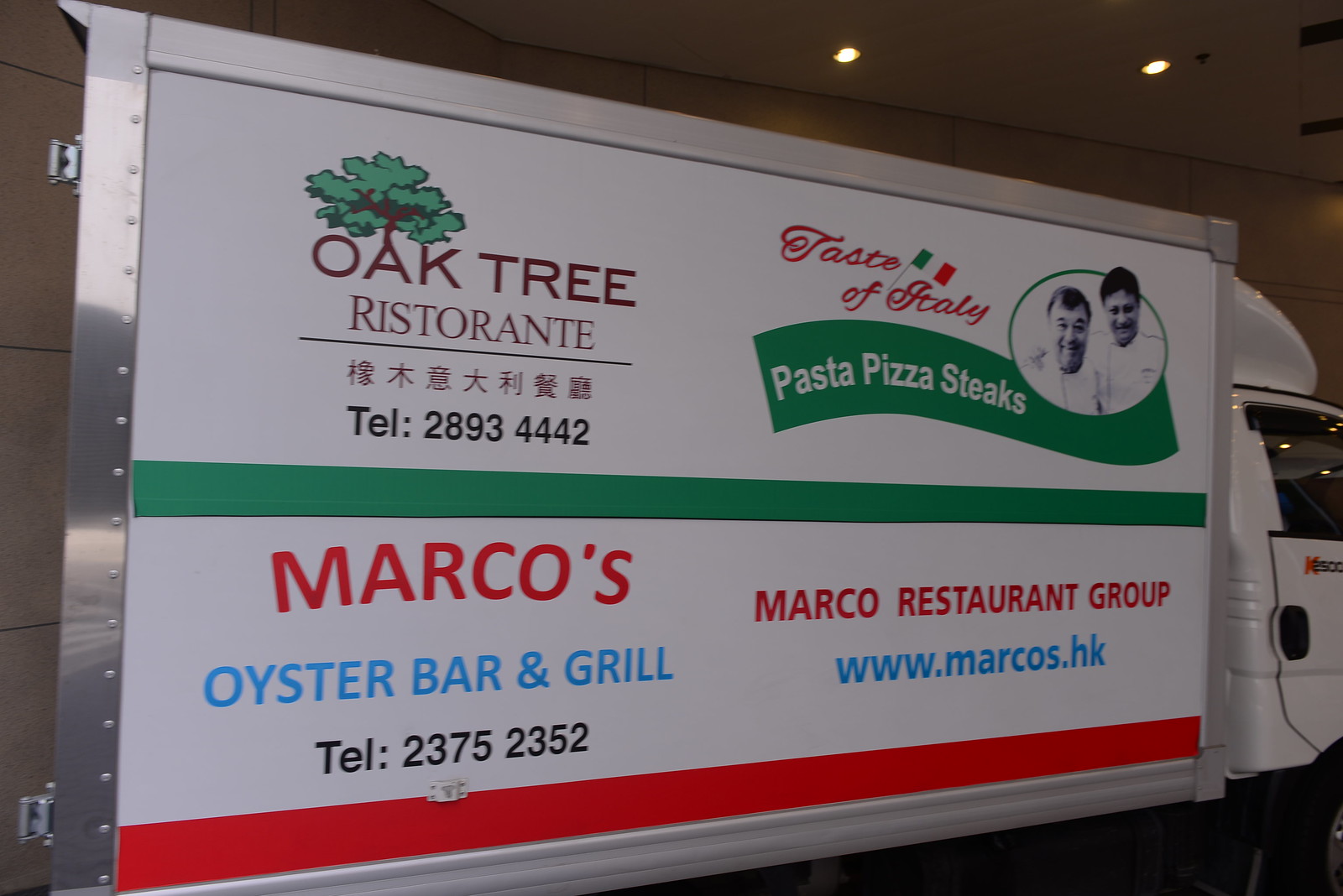The image depicts the side panel of a white box truck with detailed advertisements for restaurant establishments. The top section of the truck features the logo "Oak Tree Ristorante," with an oak tree growing out of the "A" in "Oak." Accompanying this logo is a contact number, 2893-4442, and a line of Chinese characters. To the right of this logo, in cursive red text with the Italian flag over "Italy," it states: "Taste of Italy." A black-and-white photograph of two smiling men in chef coats is centered below, alongside a green banner with white text reading "Pasta Pizza Steaks."

Below the top section, a green bar and a larger white bar span across the truck. The white bar includes "Marco's" in large red text, "Oyster Bar and Grill" in smaller blue text, and another telephone number, 2375-2352, in black. At the bottom right, it states "Marco Restaurant Group" in red text along with the URL "www.marcos.hk" in small blue text. The design is framed by bars running across the middle and bottom of the truck, creating a cohesive promotional display. The truck's cab is visible, featuring indistinguishable text under the passenger window, and the background reveals a plain, light beige building with embedded ceiling lights.